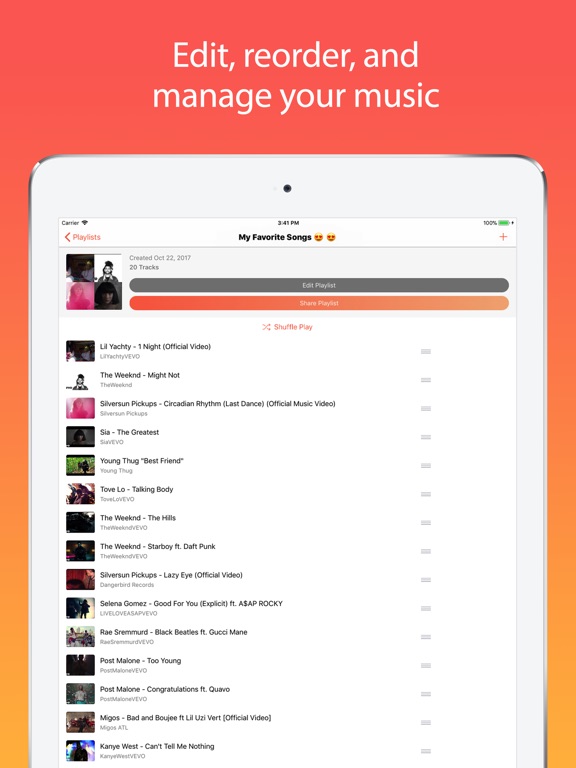This image features a smartphone screen displaying a music management interface with the options to edit, reorder, and manage your music. At the top of the screen, the heading reads "My Favorite Songs," accompanied by two emojis. Below this heading is a list of song titles in small font. Although the text is somewhat difficult to read, several song titles and artists can be discerned. The visible songs in the list include:

1. Lil Yachty - "One Night" (Official Video)
2. The Weeknd - "Might Not"
3. Giverum - "Pickups"
4. Sire - "The Greatest"
5. Young Thug - "Best Friend"
6. Tovo - "Low"
7. Talking Body - "The Weeknd"
8. The Weeknd - "The Hills"
9. The Weeknd - "Starboy" (featuring Daft Punk)
10. Silver Sun Pickups - "Lazy Eye" (Official Video)

The details of the other songs in the list are too small to be clearly read.